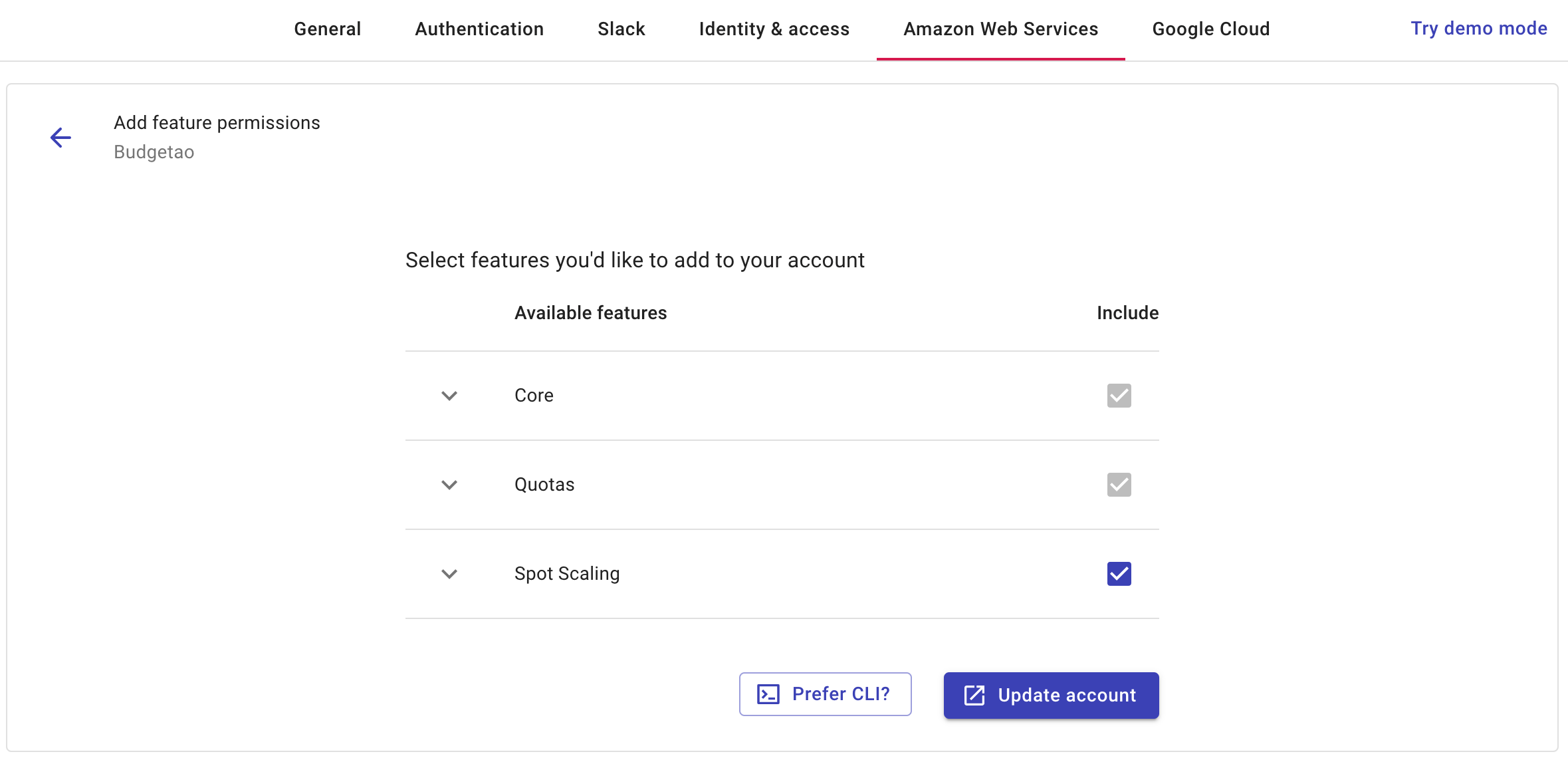On this webpage, the overall theme is primarily black and white, accented with a few colorful elements and a single red line. At the top of the page is a black-lettered menu bar, listing the sections: "General", "Authentication", "Slack", "Identity and Access", and "Amazon Web Services". The "Amazon Web Services" section is highlighted with an underlining red line. To the right of the menu, there is a gap followed by the words "Google Cloud", a space, and the phrase "Try Demo Mode" written in purple letters.

Beneath the top menu, two faint gray horizontal lines span the width of the page. On the very left, aligned under "General" in the menu, there's a purple arrow pointing left with the text "Add Feature Permissions" next to it, and below that, the words "Budget AO". 

Centrally located under the “Authentication” section, there is an instruction line reading "Select Features You'd Like to Add to Your Account." Below this, the text "Available Features" appears to the left, with the word "Include" positioned farther right. A faint gray horizontal line separates the sections.

Three expandable lines, each marked by arrowheads that point downwards, follow. The first line, labeled "Core", has a gray box with a white checkmark under the "Include" column. Underneath it, "Quotas" and "Spot Scaling" are equally formatted, each separated by faint gray horizontal lines. The "Quotas" line also has a gray box with a white checkmark under "Include", while "Spot Scaling" features a purple box with a white checkmark.

At the bottom of the image, under the "Include" column, there is a wide purple rectangle labeled "Update Account" in white letters, decorated on the left with a white outlined box and an upward-right pointing arrow. Adjacent to this purple rectangle, to its left, there is another rectangle outlined in faint purple. Its background is white with the text “Prefer CLI?” written in purple letters and a small purple icon to the left of "Prefer", consisting of a purple square with internal purple marks.